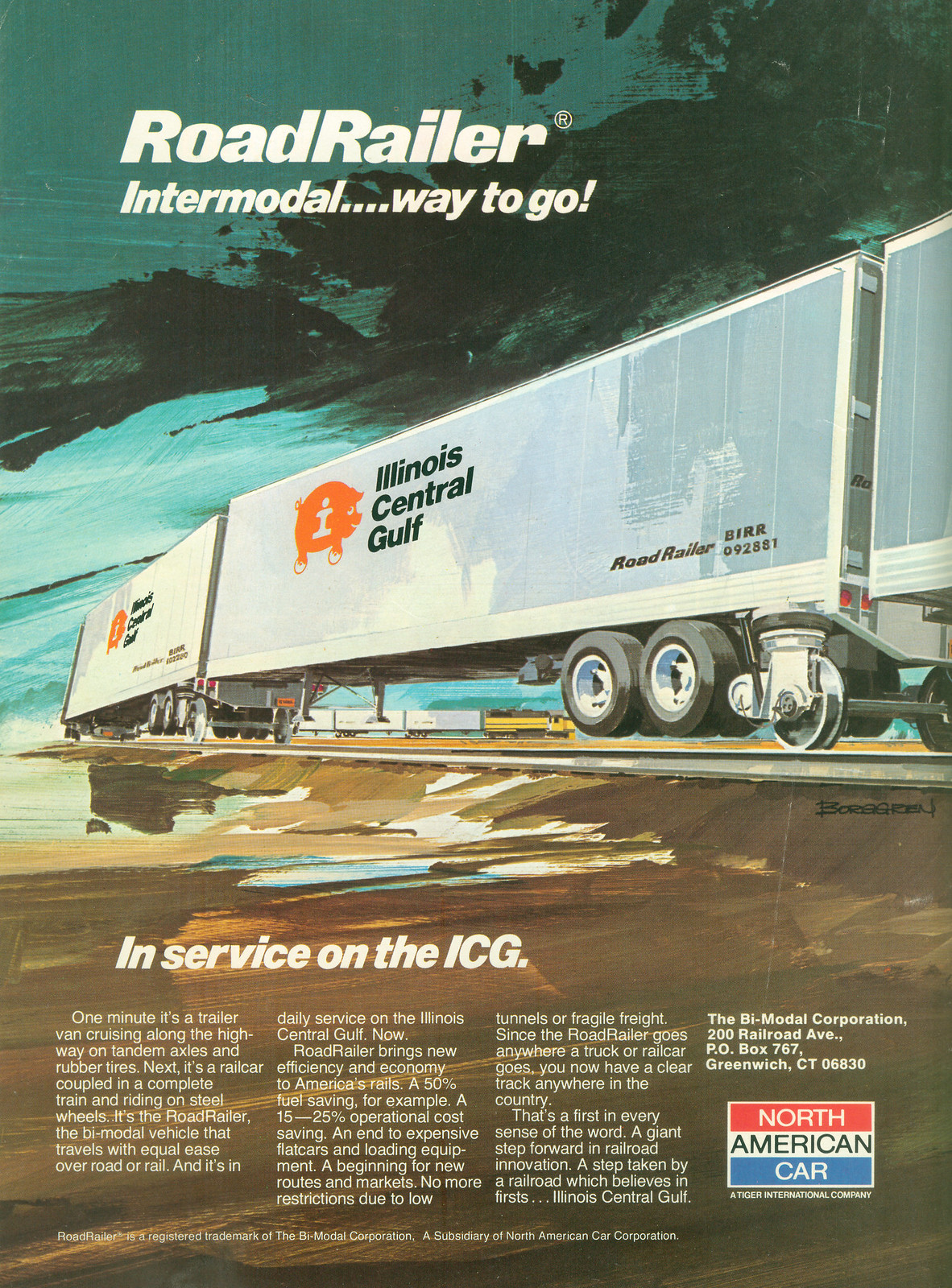This vintage-looking magazine cutout features a detailed, animated railroad advertisement from what appears to be the 70s or 80s. The colorful poster predominantly showcases a train traveling on a curved track against a backdrop that hints at forested mountains. At the top, the headline reads "Road Railer" in green letters, followed by "Intermodal, Way to Go!" in white with an exclamation point. The focal point of the ad is the train with three railway cars, notable for their dual-mode design, with one car visibly equipped with rubber tires, suggesting a bimodal capability.

Prominently displayed on the side of the train cars is the name "Illinois Central Gulf" in black letters on a white background, complemented by an orange logo with the letter "I" and the stylized image of a pig. Beneath the train cars, the text "In Service on the ICG" is printed in white against a brown background. In the bottom right corner, the text "North American Car" appears in a red, white, and blue segmented square, adding to the patriotic theme of the advertisement. The detailed illustration and vibrant colors make it clear that this train and its intermodal capabilities represent a significant innovation in modern transportation.